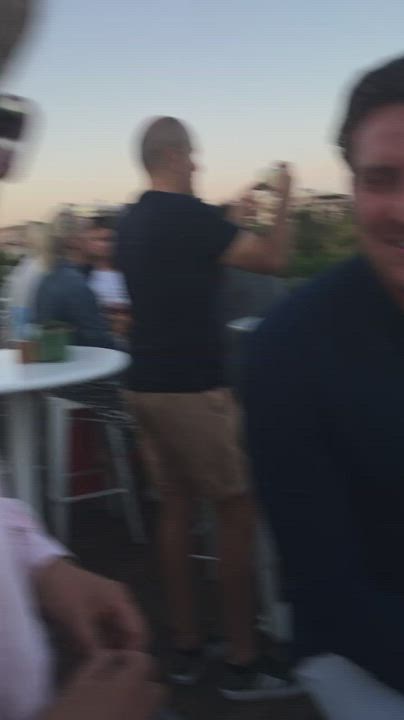This blurry color photograph captures an outdoor scene at what seems to be a restaurant or bar's deck during the evening, with the setting sun casting a gradient from light blue to orange across the sky. In the center, a bald man, possibly holding up a phone or a bottle, stands out; he's dressed in a black short-sleeve shirt, knee-length khaki shorts, and gray Adidas sneakers, facing away from a tall white circular table with a brown and green box on it. On the right, partially cut off by the frame, is a Caucasian man with brown hair wearing a dark blue long-sleeve shirt and light-colored pants. Nearby, a blurry figure in a pink shirt is prominent in the foreground. The background reveals various indistinct figures: a woman in a denim jacket and black and white bottoms, and others whose attire and features blend into the indistinct crowd. White stools and tables, along with the hazy outlines of buildings, suggest a casually bustling social setting.